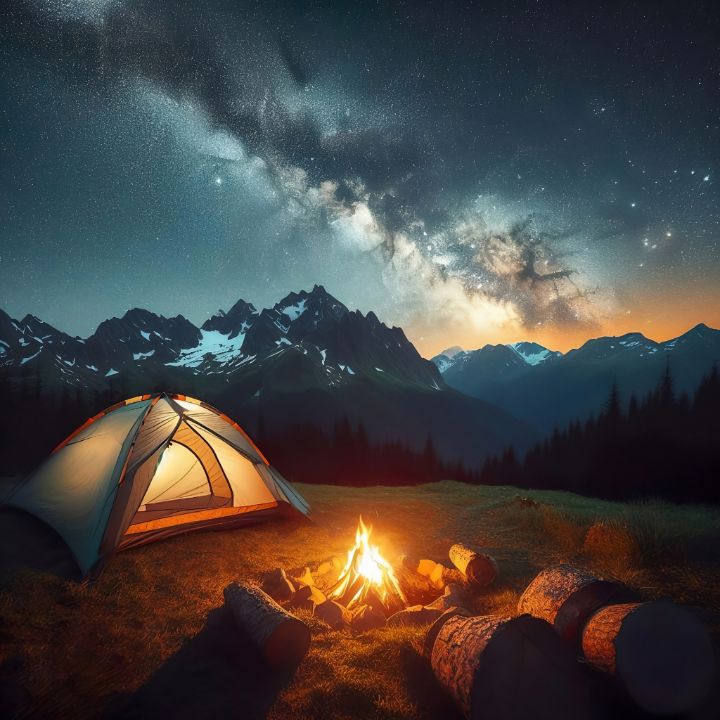This vertical rectangular image depicts a meticulously staged nighttime campsite that could easily be featured in a nature or lifestyle magazine. Central to the scene is a brown and white tent, illuminated from within, positioned near a blazing campfire. The campfire is encircled by carefully placed rocks and has a stack of burning wood at its center. Surrounding the fire are several sawn logs, serving as makeshift seating. The campsite is set in a grassy clearing flanked by towering evergreen and pine trees, suggesting a forest environment.

In the far distance, a range of snow-capped mountains looms under a twilight sky, where the setting sun casts an orange glow just behind the peaks. The remainder of the sky is clear, showcasing clusters of stars and a prominent view of the Milky Way, adding a celestial touch to the serene scene. No people are present, creating a peaceful and untouched atmosphere. The overall image, while strikingly detailed and picturesque, carries an air of artificial perfection, hinting that it may have been digitally composed or enhanced for a polished, idealized effect.